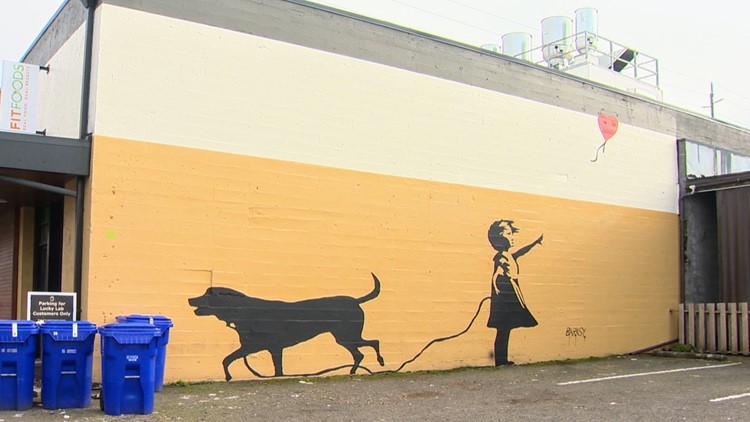This vibrant outdoor color photograph, taken in landscape orientation, captures a detailed mural painted on the exterior of a two-story building. The focal point is a whimsical scene featuring a young girl and her dog, rendered in striking black silhouette. The girl, dressed in a short outfit with her hair blowing in the wind, is positioned on the right side of the mural, looking and pointing upward toward a red balloon that has drifted into the sky, near the top of the image. She holds a leash, leading to a dog depicted in profile, walking toward the left side of the frame, seemingly in the opposite direction of its owner.

The mural's backdrop is divided into a light orange color at the bottom, reminiscent of brick, transitioning to a cream color at the top. The building's fencing structure, visible at the roofline, is painted white, contrasting with a gray section just below it. On the left-hand corner of the scene, four blue garbage cans are neatly arranged. Adding a personal touch to the setting, a doorway on the right side bears a sign reading, "Parking for Lucky Lab customers only." The photographic style of realism imbues the mural with a dynamic, life-like quality, creating a captivating visual narrative.